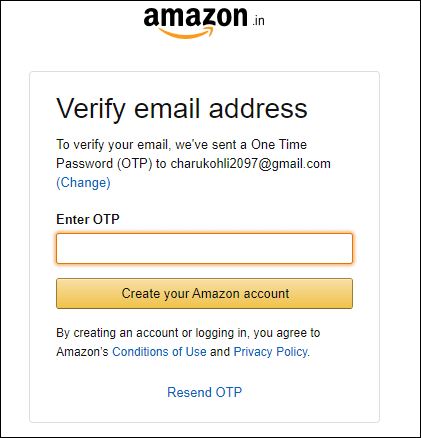This image is a screenshot of the email address verification step during the account sign-up process on the Indian version of Amazon (amazon.in). The layout is almost a perfect square, framed by a thin, one-pixel black line. Inside this boundary is the familiar Amazon logo, featuring the iconic smile that extends from the "A" to the "Z".

At the top center, the text "Verify email address" is prominently displayed in the largest font size. Beneath it, a smaller text sentence reads: "To verify your email, we've sent a one-time password (OTP) to charakoli2097@gmail.com." Adjacent to this information, a blue text link offers the option to change the email address.

Below this, the form instructs users to "Enter the OTP," encircled by a glowing orange line that highlights the input field. Directly under the field, an orange button is labeled "Create your Amazon account."

At the bottom of the form, additional text states: "By creating an account or logging in, you agree to Amazon's Conditions of Use and Privacy Policy," with "Conditions of Use" and "Privacy Policy" presented as clickable blue text links. A final blue text link labeled "Resend OTP" is positioned at the very bottom, offering the option to receive another one-time password.

The entire layout is meticulously designed to guide the user through verifying their email address as part of the Amazon account sign-up process.